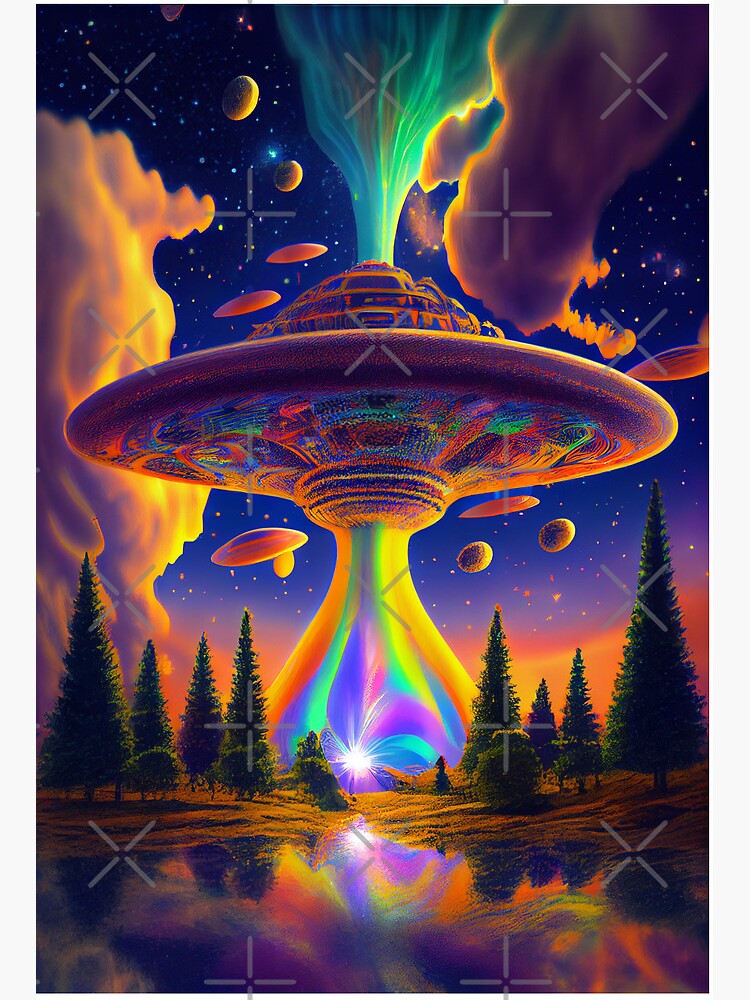This artwork, potentially computer-generated or hand-done in colored pencil or chalk style, vividly captures a psychedelic scene with a UFO of 1940s-50s saucer design. The spaceship features a large central disc with smaller, stacked discs on top and a slight bubble protruding from the bottom. Its surface is adorned with swirling, fabric-like patterns in greens, reds, blues, and yellows, giving it a textured appearance. Multicolored beams and goo, resembling toothpaste and in vibrant hues like oranges, extend from the bottom, while smoky green to blue-green vapor emerges from the top.

The UFO hovers just above a tree-lined landscape, featuring tall, pointy fir trees, a rustic lake or pond reflecting the spaceship's kaleidoscopic colors. The ground is covered with yellowish grass, and the water mirrors the ship in its vibrant shades.

Surrounding the spacecraft is a night sky transitioning from dark black to a gradient of blue, dotted with various stars and planets in yellow and blue. There are also peculiar objects resembling pink oysters and yellow meatballs scattered around. To the left and top-right, marshmallow-like clouds extend upwards, adding to the artwork's 70s-style, lava lamp aesthetic. Above the spaceship, these clouds further morph into a green vapor trail, merging into the night sky, completing the surreal and fantastical scene.